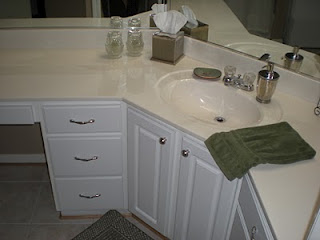The image depicts a simple and unadorned bathroom with a functional yet modest design. The bathroom features white cabinetry with basic chrome handles, which lend a minimalist touch. The sink is set into a clipped corner, reducing sharp angles for a softer look. The countertop is a warm-toned white stone marble, providing a subtle contrast to the cooler white of the cabinets.

Notably, the cabinetry includes a designated vanity area with space for a chair, allowing for comfortable seating and use. Flanking this space are drawers ideal for storing makeup and other personal items. The room features green accents, with a green hand towel and a matching rug, bringing a cohesive color scheme to the space. The countertop hosts a few decorative items, including glass jars, a tissue dispenser, a soap dish, and a chrome pump-style hand wash dispenser, adding both functionality and a touch of elegance.